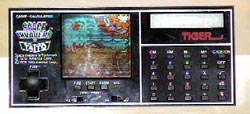The image appears to depict a screenshot of a handheld gaming console, specifically one that resembles the classic "Tiger" electronic games from the 90s. The console itself is black and rectangular, with a distinctive "Tiger" logo in red at the top center. Above the logo, there is a small white rectangular box, likely displaying game information. The left half of the console features a brown directional pad (D-pad) in the shape of a plus sign (-), while the center and right side include various smaller buttons arranged in a grid-like pattern, also bearing white text that is difficult to read. The screen of the console showcases a game interface: the top portion features a spray-painted blue color set against a black background, and the bottom half displays a series of five rows of squares or tabs with indistinct characters. The left side of the screen includes the text "Space Invaders" with additional smaller, hard-to-read writing below it. Overall, the left and right sections of the console are bordered in brown, with the rest accented in black and white.